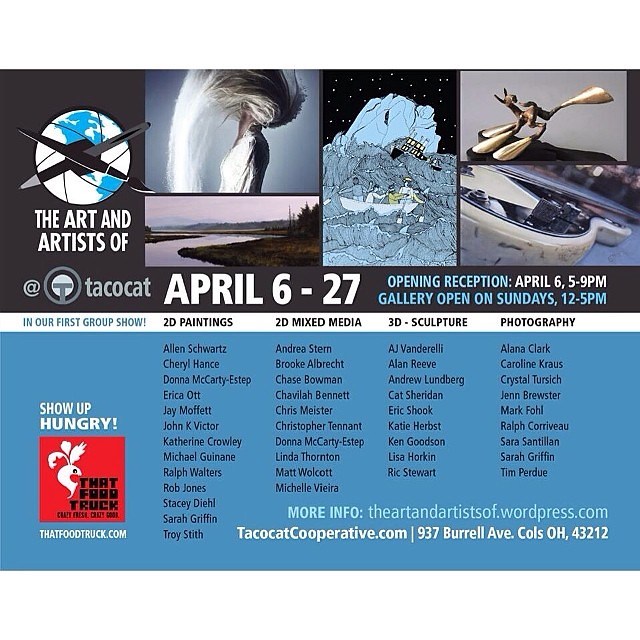The promotional banner advertises an art exhibition titled "The Art and Artists of Taco Cat," displayed against a grey top half transitioning to a light blue bottom half. The top section features four distinct images: a woman with her hair fanning out, a river, a drawing of a boat on a choppy sea, and a sculpture. Above these images, the text reads "The Art and Artists of Taco Cat" with a globe icon, a pencil, and a paintbrush illustrating creativity. Key event details are prominently displayed in white and blue text, announcing "April 6th through the 27th" and "Opening Reception April 6th, 5 to 9 p.m., Gallery open on Sundays 12 to 5 p.m."

A white banner separating the two sections highlights the types of artwork on display: "2D paintings, 2D mixed media, 3D sculpture, and photography." The bottom blue section lists numerous artists' names in black text across four columns and includes an invitation written in white to "show up hungry," indicating that food will be available, likely provided by "That Food Truck" (referenced with a logo and URL: thatfoodtruck.com). Additional information is provided at the bottom right, with website addresses for more details: theartandartistsof.wordpress.com and tacocatcooperative.com, along with a location noted as 937 Burrell Avenue, Columbus, Ohio 43212.